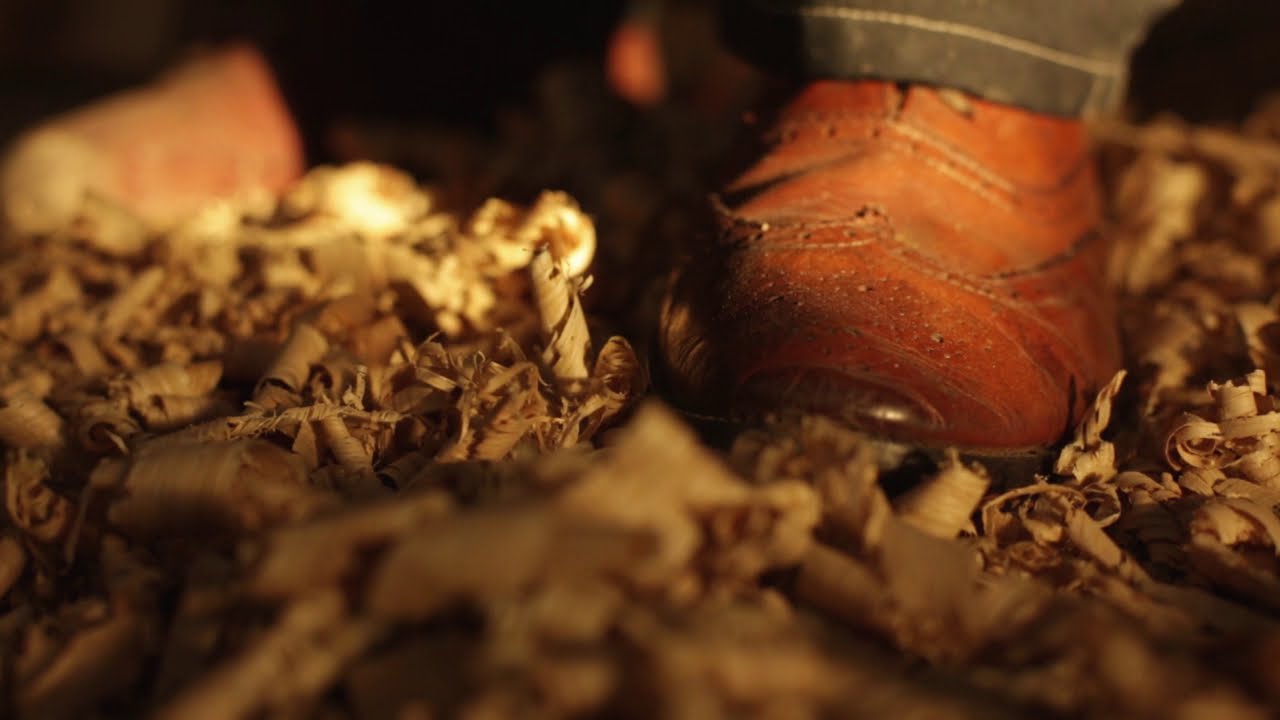In this close-up image, a man's right foot, wearing a worn, brown leather dress boot with decorative stitching, pointed toe, and burnished dark brown tip, is stepping into a pile of light brown wood shavings. The boot features intricate wingtip designs and small punched holes, indicative of classic craftsmanship. The man's dark gray cuffed jeans are visible, ensuring a clear view of the shoe’s detailed design. The majority of the image is dominated by the scattered wood shavings, which are clear in the center and blur towards the bottom. The background is a stark dark contrast, suggesting the photo might be taken outdoors at night, giving an artistic focus on the shoe and the texture of the wood shavings. There is no text visible in the image.